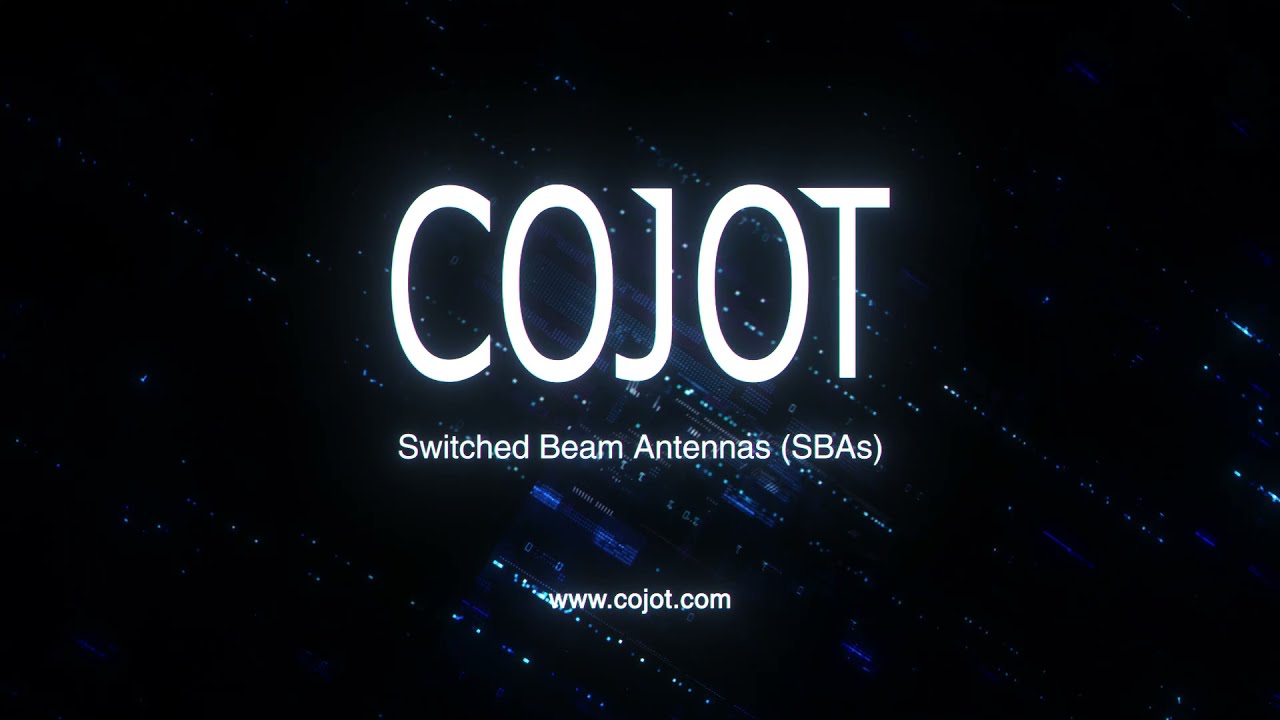In the image, a black background is accentuated by streaks of light and abstract patterns, including dim blue and white lights that suggest a futuristic or high-tech design. Diagonal lines, resembling raindrops or light streaks, traverse the image, converging at different angles and creating a dynamic sense of movement. Central to the composition is large white text in all capital letters reading "COJOT." Beneath it, smaller white text states, "Switched Beam Antennas" with the abbreviation "S-B-As" in parentheses. At the bottom of the image, a white URL, www.cojot.com, is displayed.